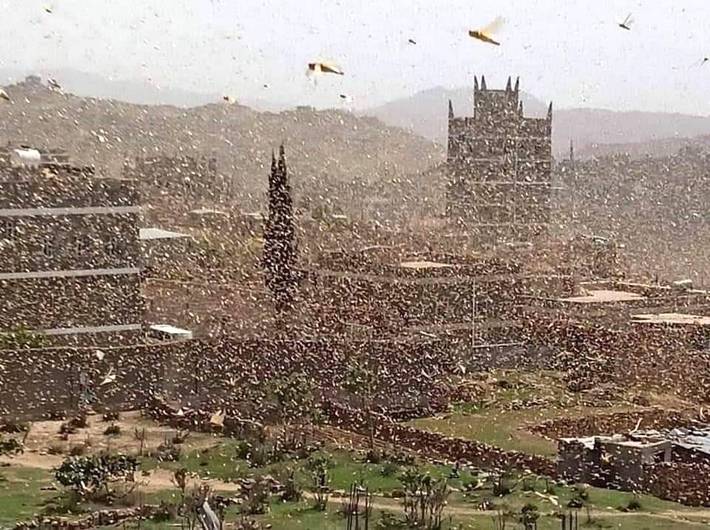The image captures a wide-angle aerial view, akin to a drone's perspective, of what appears to be an ancient or medieval city, possibly a castle in Europe, characterized by its very old architecture. The city is enveloped in a swarm of flying insects, potentially locusts or dragonflies, moving predominantly in a direction akin to the nine o'clock position. The scene is shrouded with numerous white specks, which could be artifacts or suggest a blizzard-like condition, although no snow is visible. This haze of insects covers the entire scene, obscuring the detailed view of the large buildings, parks, and trees below. The background reveals large, dimly seen mountains under a gray, cloudy sky, with the insect horde contributing to the overall obscurity. Near the base of the image, patches of green grass and intertwining paths are discernible, providing a stark contrast to the overwhelming presence of the insects above.